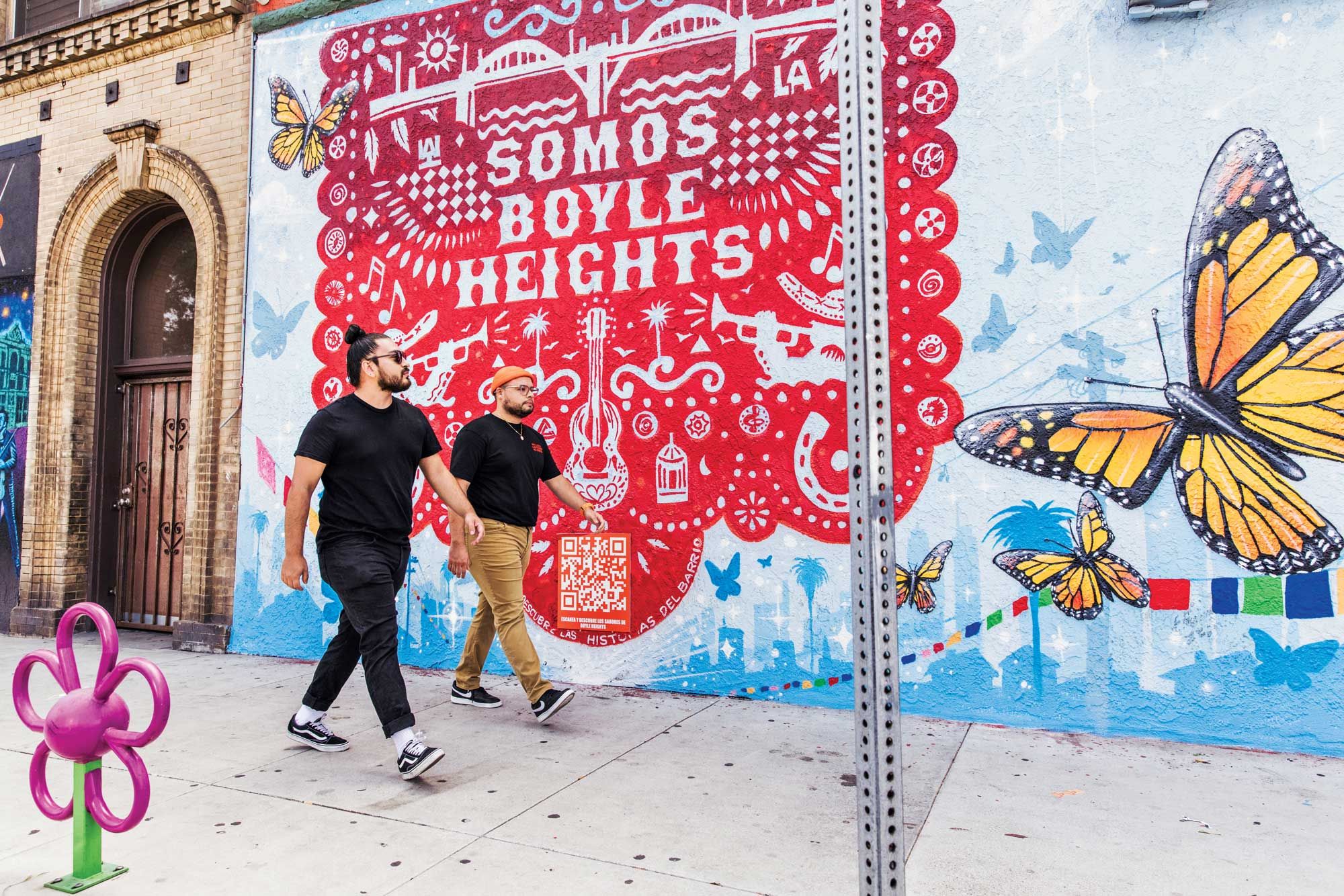This photograph captures a vibrant street scene in Boyle Heights, California. Two men are walking side by side, both wearing black t-shirts. The man on the left is dressed entirely in black, with black jeans, Vans sneakers with white socks, and dark sunglasses, his black hair styled in a bun. The man on the right wears an orange beanie, glasses, a black t-shirt, khaki pants, and black and white Nike sneakers. They are walking past a vividly painted mural that reads "Somos Boyle Heights." The mural's design highlights the cultural richness of the Hispanic community with an array of large, eye-catching butterflies in shades of tans, oranges, and bright yellow, some appearing as silhouettes. Additionally, there are elements of blue palm trees and a striking purple daisy-like plastic flower with a green stem adding to the colorful and culturally rich atmosphere of the scene. Neither of the men is looking at the photographer, focusing instead on the path ahead.